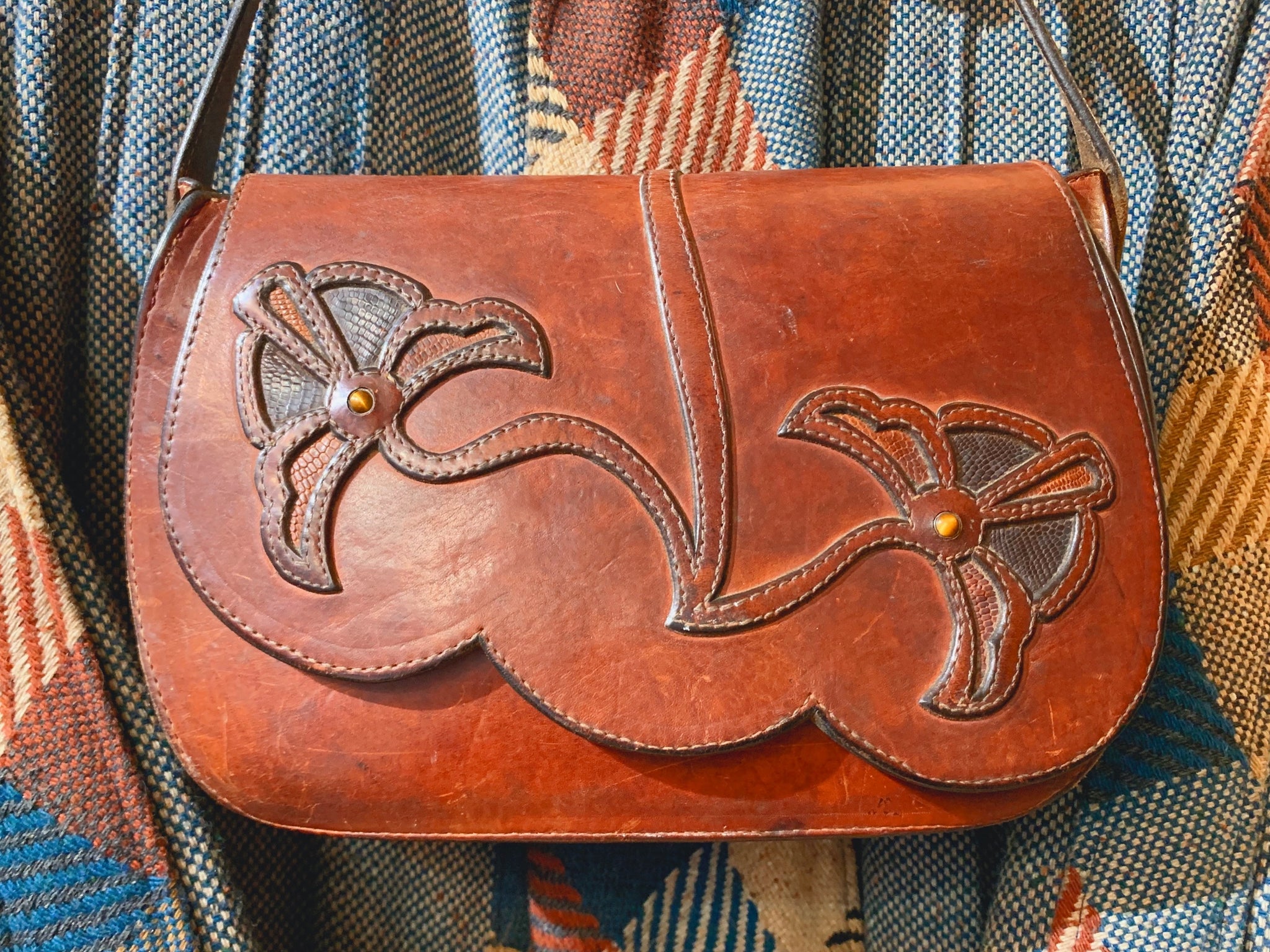The image features a medium brown leather purse adorned with intricate details. The purse displays a raised leather design resembling winged shapes or crab claws, with an ornate floral motif across its scalloped-edged flap, which consists of three large scallops. Two prominent shapes on the flap, suggestive of petals or wings, create a symmetrical pattern connected by a central seam. The leather design elements are accentuated by different colored leather inlays and a brass pin holding them together. Two black and brown straps are visible, adding to the bag's rustic charm. The purse is set against a folded, draped fabric background composed of a woven, patchwork quilt-like pattern featuring alternating squares of yellow, blue, gray, brown, and vivid touches of white and orange, reminiscent of a prairie or Indian style. The intricate interplay of colors and textures between the purse and the fabric background creates a visually striking composition.